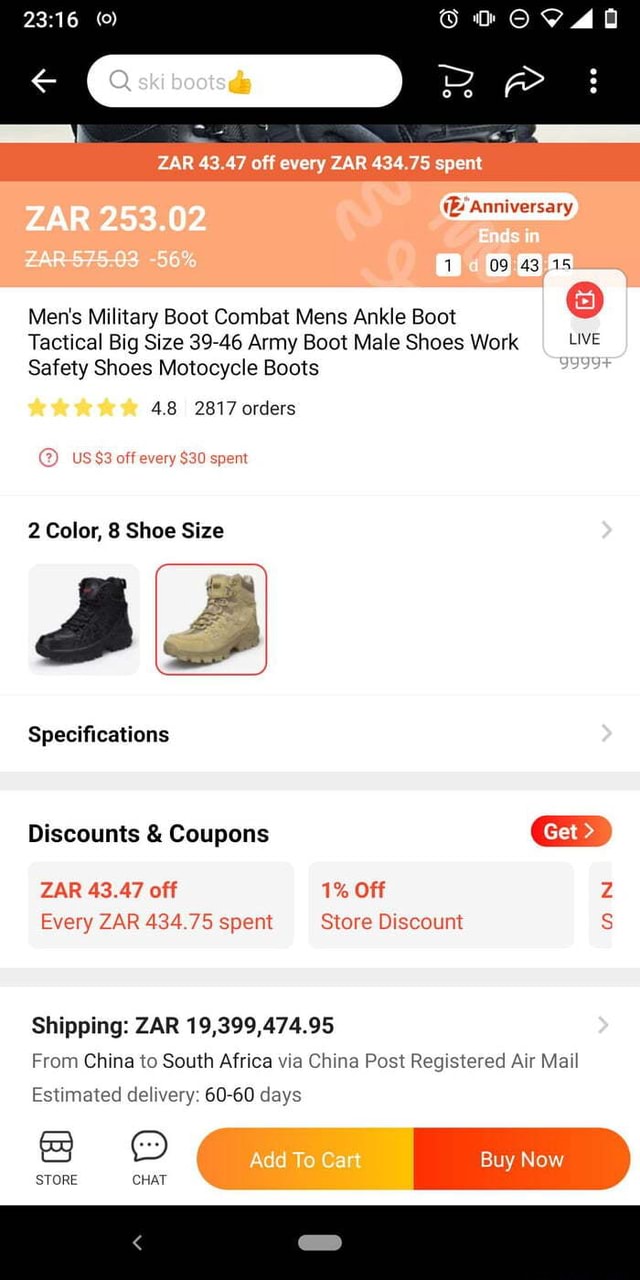Screenshot of a Mobile Webpage Displaying Shoe Sale Details:

The screenshot shows a mobile webpage focused on selling shoes, likely taken from a tablet or smartphone. The device status bar indicates the time is 23:16 in military time. There are several icons, including an unrecognized notification, an alarm set icon, a vibration mode icon, a “Do Not Disturb” icon, a nearing depleted battery indicator, and a strong wireless signal icon.

In the browser’s URL bar, there is a white left-pointing arrow. Next to it is a search bar with the text "ski boots" accompanied by a yellow-orange thumbs-up icon. On the far right, there is a shopping cart icon, a right-pointing arrow for forwarding, and three vertical ellipses for additional settings.

Below this, there is an orange banner with bold white text stating: "ZAR 43.47 off every ZAR 434.75 spent." Following this banner is a lighter orange section displaying "ZAR 253.02," "ZAR 575.03," and a "-56% discount." On the right side, there is a red button labeled "Anniversary 12" with a dark gray background and the word "ENDS" below it, followed by a countdown timer showing "1 day, 9 hours, 43 minutes, and 15 seconds."

In the main content section, two boots are displayed—one black and one tan. The text reads: "Men's military boot, combat, men's ankle boot, tactical, big size, 39-46, army boot, male shoes, work, safety shoes, motorcycle boots." The product has a rating of 5 out of 5 stars based on 2,817 orders. There is a "?" icon in a circle with the text "list $3 off every $30 spent" under it, and below that, the word "qualifications" in bold black text.

Above the boots, it states "$2 each shoe size" with "tan" being the selected color. The page also shows discount coupons offering "ZAR 43.47 off every ZAR 434.75 spent" and "$1 off." On the right is a circular button labeled "GET" with an arrow.

At the bottom, the shipping details are presented as: "ZAR 19,399,417.95 (actually $19,399,474.95) from China to South Africa via China Post registered air mail, estimated delivery 60 to 90 days." There are two buttons: a white-texted orange button labeled "Add to Cart" and a dark orange button labeled "Buy Now." The screen also features a store icon and a chat icon.